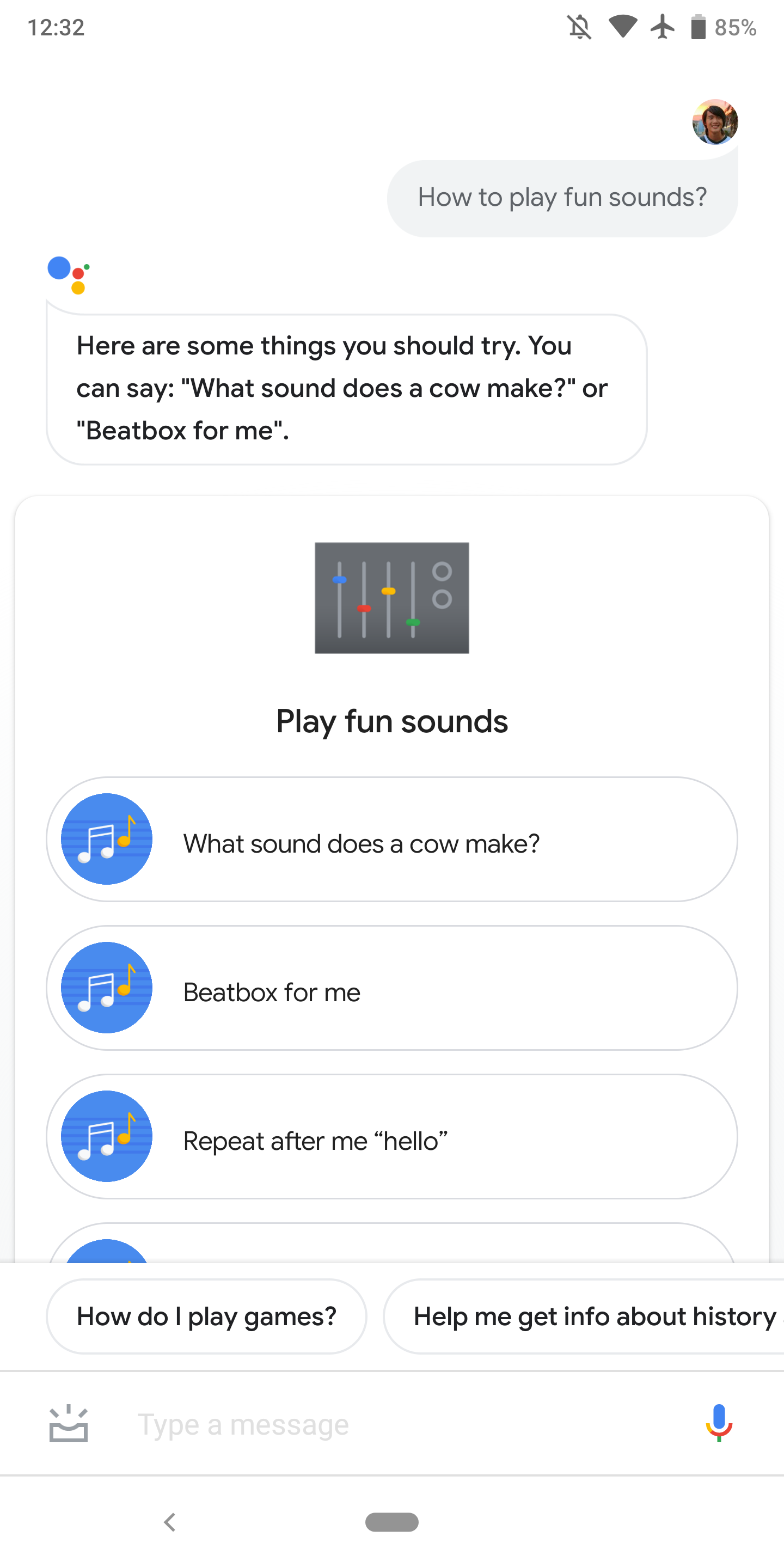This image is a screenshot captured from an Android phone in portrait orientation, distinctly taller than it is wide, set against a white background without prominent borders. 

In the top left corner of the screen, the time is displayed as 12:32. To the right of the time, several status icons are visible: a silent mode icon represented by a bell with a line through it, a fully lit Wi-Fi signal strength icon, an airplane symbol indicating airplane mode is active, and a vertical battery icon showing a charge level of 85%.

Below the status bar, there is an avatar featuring a woman standing in front of a sunset, accompanying a gray text bubble that reads, "How to play fun sounds." The subsequent response from Google Assistant follows, marked by its multicolored icon (blue, green, red, and yellow circles). Google Assistant suggests various interactive prompts with the message, "Here are some things you should try. You can say, 'What sound does a cow make,' or 'Beatbox for me.'"

Further down, a white box with a thin gray border contains a stylized image of a synthesizer in black, adorned with levers in Google's signature colors. This section is titled "Play fun sounds." Below it, four blue circles with musical note icons introduce additional options; each circle includes a text bubble with prompts such as "What sound does a cow make," "Beatbox for me," and "Repeat after me: hello." There are also suggested questions listed, like "How to play games" and "How to get info about his...".

The overall composition clearly highlights the interactive features and user interface elements of Google Assistant within the Android operating system.